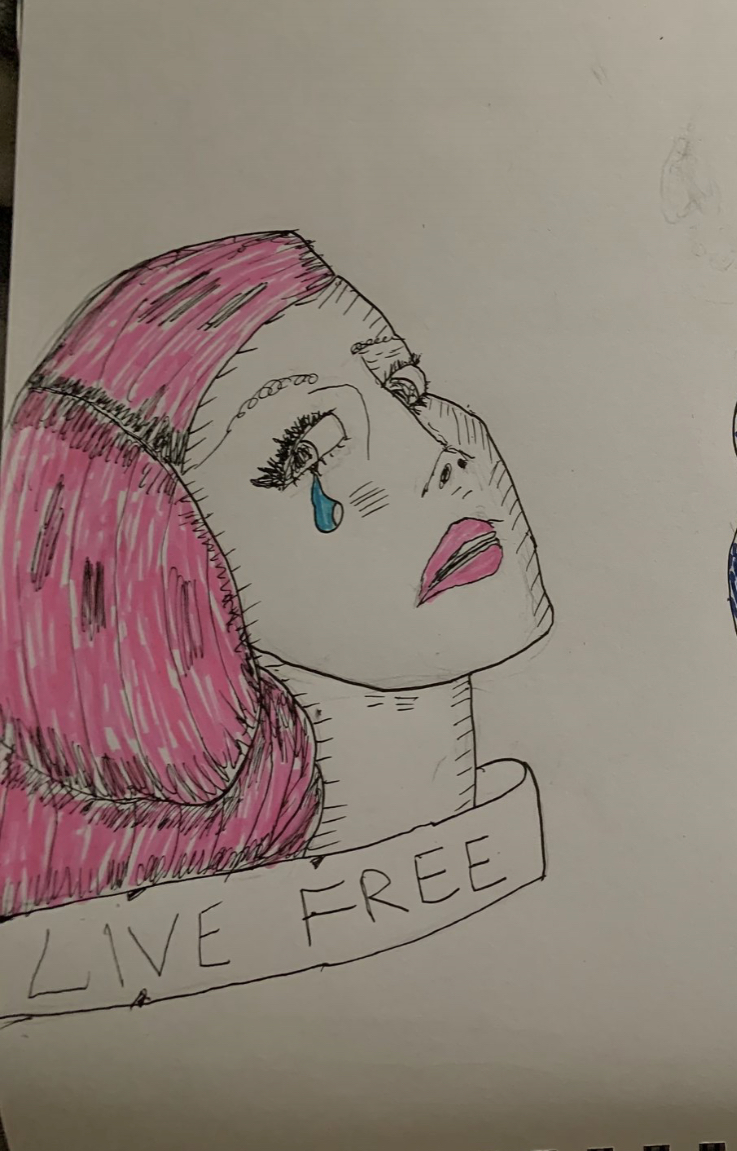This detailed pen and felt-tip illustration captures the melancholic visage of a young woman. The focal point of the artwork is her face, drawn with simplistic yet expressive lines. Her eyes shed a single, vivid blue tear. Her lips, notably pink, stand out against the otherwise uncolored features of her face, including her slim nose, visible nostrils, eyelashes, and eyebrows. Her bright pink hair is combed back, framing her face and extending down to reveal a slender neck that remains devoid of color. Adding an element of depth and symbolism, a ribbon-like logo encircles her neck, originating from the back of her hair, with the poignant inscription "Live Free" emblazoned on it. The entire piece is crafted on a plain sheet of paper, utilizing a blend of pens and felt-tip markers, highlighting the emotional and artistic expression of the subject.